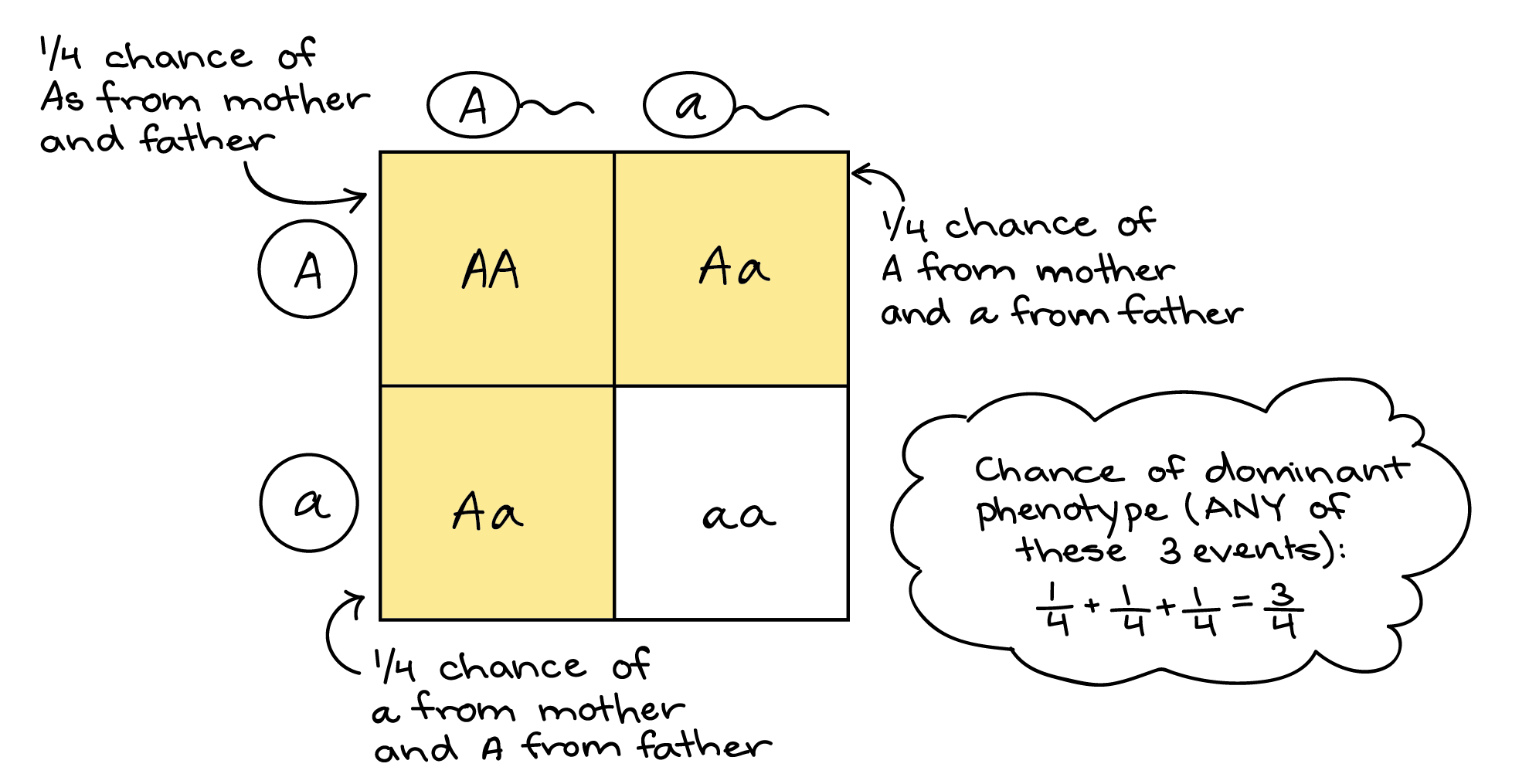This image depicts a detailed Punnett square, commonly used in genetics to predict the probability of offspring inheriting certain traits. The Punnett square consists of a 2x2 grid showing combinations of alleles from the parents. The upper left square displays two capital A's (AA) and the upper right square shows a capital A and a lowercase a (Aa). The lower left square also contains a capital A and a lowercase a (Aa), while the bottom right square has two lowercase a's (aa). All squares except the bottom right are colored yellow, indicating the dominant phenotype. Each quadrant of the grid represents a 1/4 chance of occurrence if these alleles are passed down from the mother and father. Additionally, a cloud thought bubble in the lower right notes, "Chance of dominant phenotype: any of these three events (AA, Aa, Aa) equals 3/4." This image is likely from a scientific textbook, illustrating the probability of inheritance in genetics.